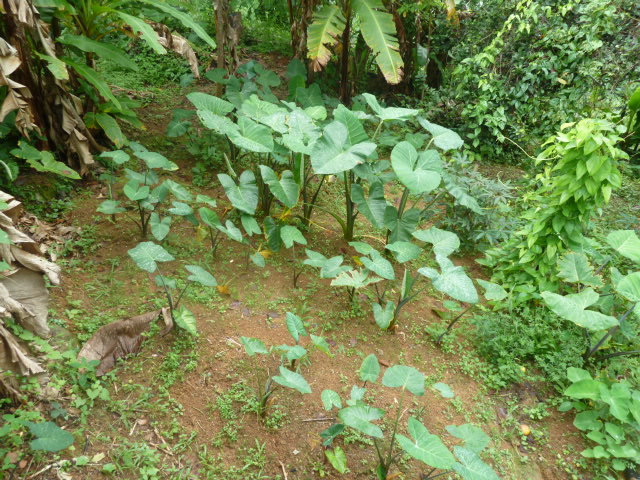The image depicts a lush, outdoor scene focused on an area of brown dirt with scattered green plants emerging from it. Dominating the center are several plants featuring large, heart-shaped leaves that resemble elephant ears, standing at about knee height. These central plants are somewhat spaced apart, allowing patches of the ground to be visible beneath them. Surrounding this central cluster, the scene is filled with dense, varied greenery. On the right-hand side, there are shorter bushes with bushy green leaves, interspersed with plants that have more delicate, shorter leaves. In the background, particularly at the top of the image, a thicket of leafy plants features long, palm-like structures that provide a tropical ambiance. Additionally, some withered brown leaves are visible towards the left side of the image, adding to the overall rich vegetation and earthy tones present throughout the scene.